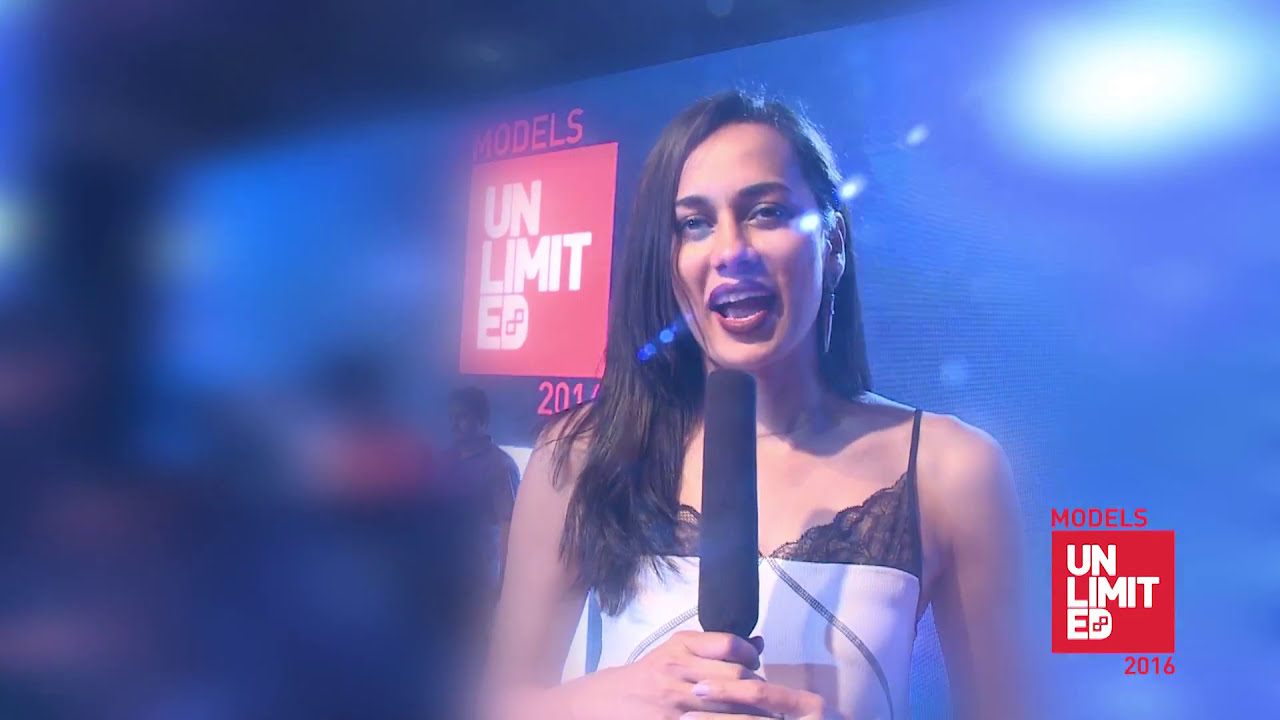In the image, a young woman with long brown hair and a tanned complexion is centered, holding a large microphone in her right hand and speaking into it. She has dark hair and wears a white shirt with black lace detailing. The event backdrop prominently displays the logo "Models Unlimited 2016" in an orange and white font, with the text appearing both in the background and the bottom right corner of the image. The scene also features a blurred background with indistinct figures, suggesting other activity at the event. Bright lights from the top right create glares, emphasizing the action nature of the shot, as the woman appears engaged in reporting or interviewing at what looks like a fashion or modeling event.